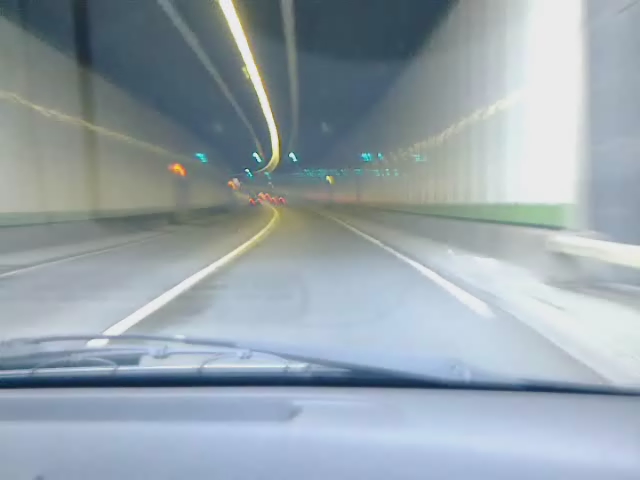The image is a photograph taken from inside a moving car at night, likely from the passenger's side perspective. In the foreground across the bottom of the photo, part of a light gray dashboard is visible, along with a windshield wiper blade lying flat on the left side. There is a faint square shadow on the left side of the image.

The car appears to be on a road with tall, white, noise-barrier walls or tunnel walls on either side, and a guardrail before the wall. The headlight reflections create a distorted effect, turning individual lights into trails. A prominent light trail runs across the center of the image, contributing to the surreal atmosphere.

In the scene ahead, you can see reflective yellow and white highway stripes glowing from the headlights, contributing to an illusion of another road above, likely a reflection in the windshield. Farther down the road are red taillights of three vehicles, receding into the distance. Green highway road signs and lights can be seen in the distance, situated in the middle of the photo. The overall scene hints at the car approaching a tunnel, with its two lanes and central lighting running along the ceiling.